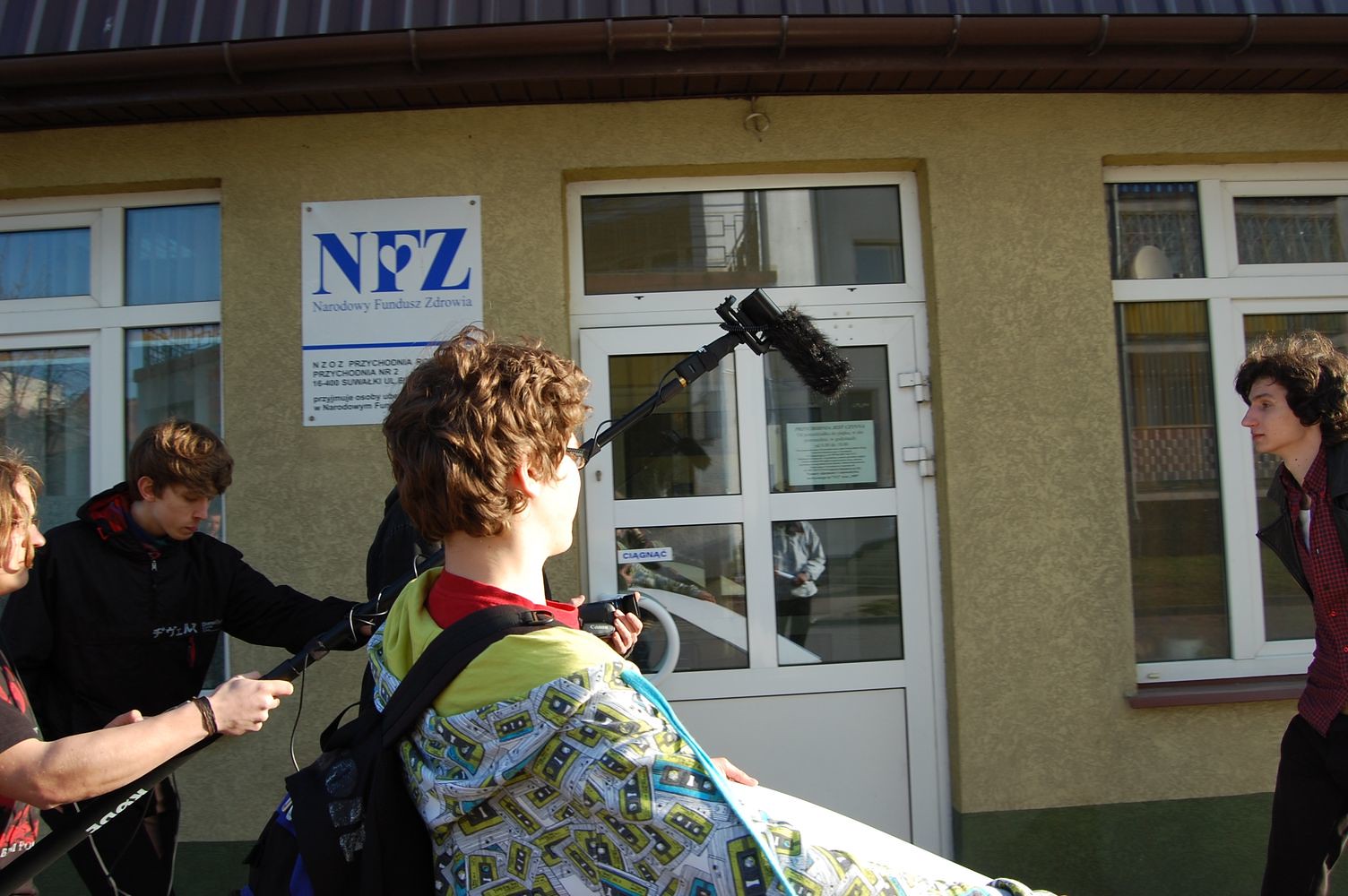In front of a tan building with a metal roof and large glass-panelled doors marked by a sign that says "NFZ" in an unknown language, a young person with medium-length curly brown hair and glasses is being interviewed. They stand near the entrance, wearing a distinctive sweatshirt adorned with cassette tape designs and carrying a backpack. In front of them, a young interviewer clad in a hoodie and backpack holds a microphone, while two other young men operate a boom microphone, capturing the exchange. Nearby, another young man in a red button-up shirt and black pants walks towards the scene. Despite the presence of the recording equipment and the interviewers' focus, the subject of the interview appears unfazed. The overall setting suggests this might be taking place outside a school building, with everyone involved appearing to be in their late teens to early twenties.